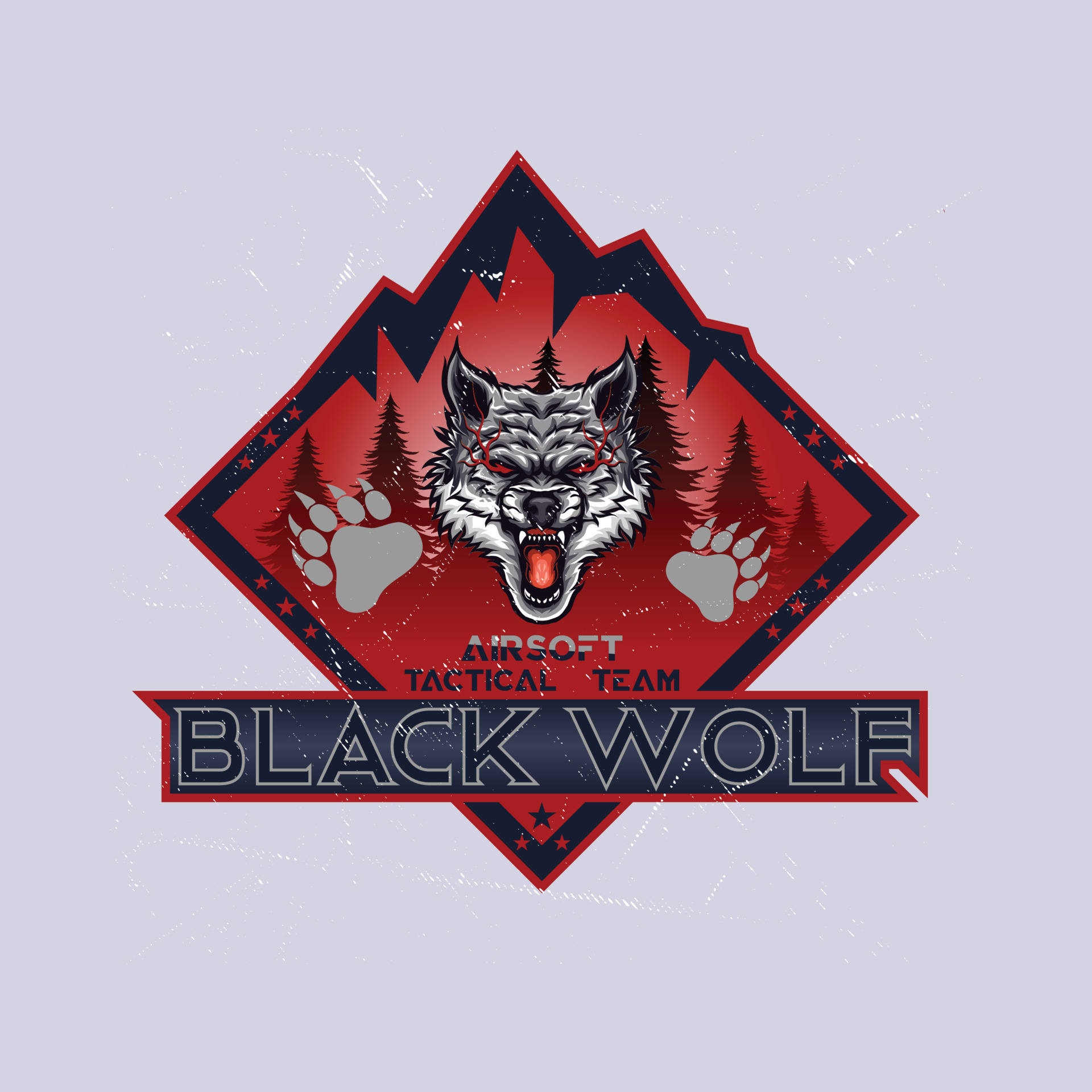The detailed logo features a menacing wolf at its center, depicted in shades of gray and white, with its mouth open wide to reveal sharp, white teeth, a red tongue, and vivid red gums. The wolf's eyes are striking, with blood or lightning-like veins emanating from them, adding to its fierce appearance. Its ears are outlined in gray, with blue and black details at their centers. Below the wolf's head, two paw prints are stamped, emphasizing its predatory nature.

The backdrop showcases a dark and foreboding wilderness with black and red trees, creating a gradient that intensifies the ominous atmosphere. Scattered across this backdrop are numerous stars: three at the bottom left, two at the center, three at the bottom right, three at mid-left, and three at mid-right, all surrounded by a zigzag pattern embroidered in blue. The entire image is outlined in red, providing a robust frame to the design.

Below the wolf's head, the phrase "Airsoft Tactical Team" is inscribed in a bold and assertive font, and under this, another rectangular sign outlined in red contains the words "Black Wolf" in black letters, set against a blue and black background. The setting appears to be a square or diamond-shaped badge, perfect for an Airsoft team's logo, characterized by its vibrant red and navy blue color scheme and striking, vectorized design elements.